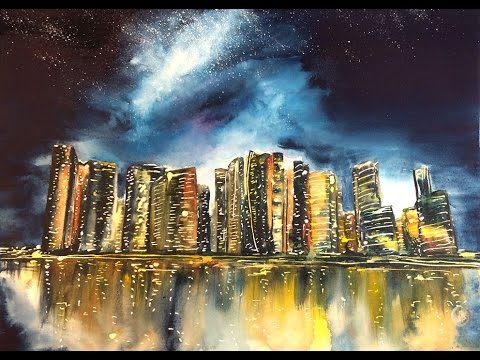This image is a detailed watercolor painting of a night-time city skyline. The scene features an array of tall skyscrapers stretching across the canvas from left to right. Each building is illuminated with lights from the windows, emitting hues of yellow, red, and subtle maroons, standing in contrast against their dark structures shaded in blacks and grays. The vivid color scheme adds warmth to the painting, while cooler tones dominate the night sky above. In the sky, faint stars twinkle amidst a mixture of cloud-like streaks in light blues, purples, and dark blues, blending seamlessly into the dark blue to black expanse of the night. A curious detail is the faint appearance of what looks like wolf's eyes within the brighter aura surrounding the city, adding a surreal touch. Below the skyline, a body of water perfectly mirrors the illuminated buildings, capturing their glowing reflections vividly, which dominate the lower half of the painting. The result is a mesmerizing and luminous portrayal of a bustling urban landscape at night.